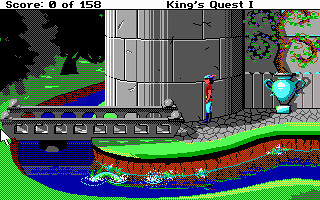This is a screenshot from the 8-bit video game King's Quest 1, highlighting a static scene with detailed pixel art. The upper section of the image displays a thin white border with the text "score: 0 of 158" on the left and "King's Quest 1" on the right. Below this header, the primary scene depicts a medieval castle situated behind a gray stone bridge that extends over a dark blue moat. Green grass surrounds both sides of the moat, integrating seamlessly into a swirling pattern.

To the left of the bridge are black and gray trees, adding to the scene's depth. On the right side of the bridge, standing motionless, is a character resembling a bard. He wears a sky-blue cap with a red feather, a red shirt, blue pants, and black knee-high boots. Adjacent to him is a large blue vase or chalice with a plant emanating from it, its leaves and branches forming a curling pattern. The whole scene is rendered in a distinctly old-school, pixelated style, typical of early video games.